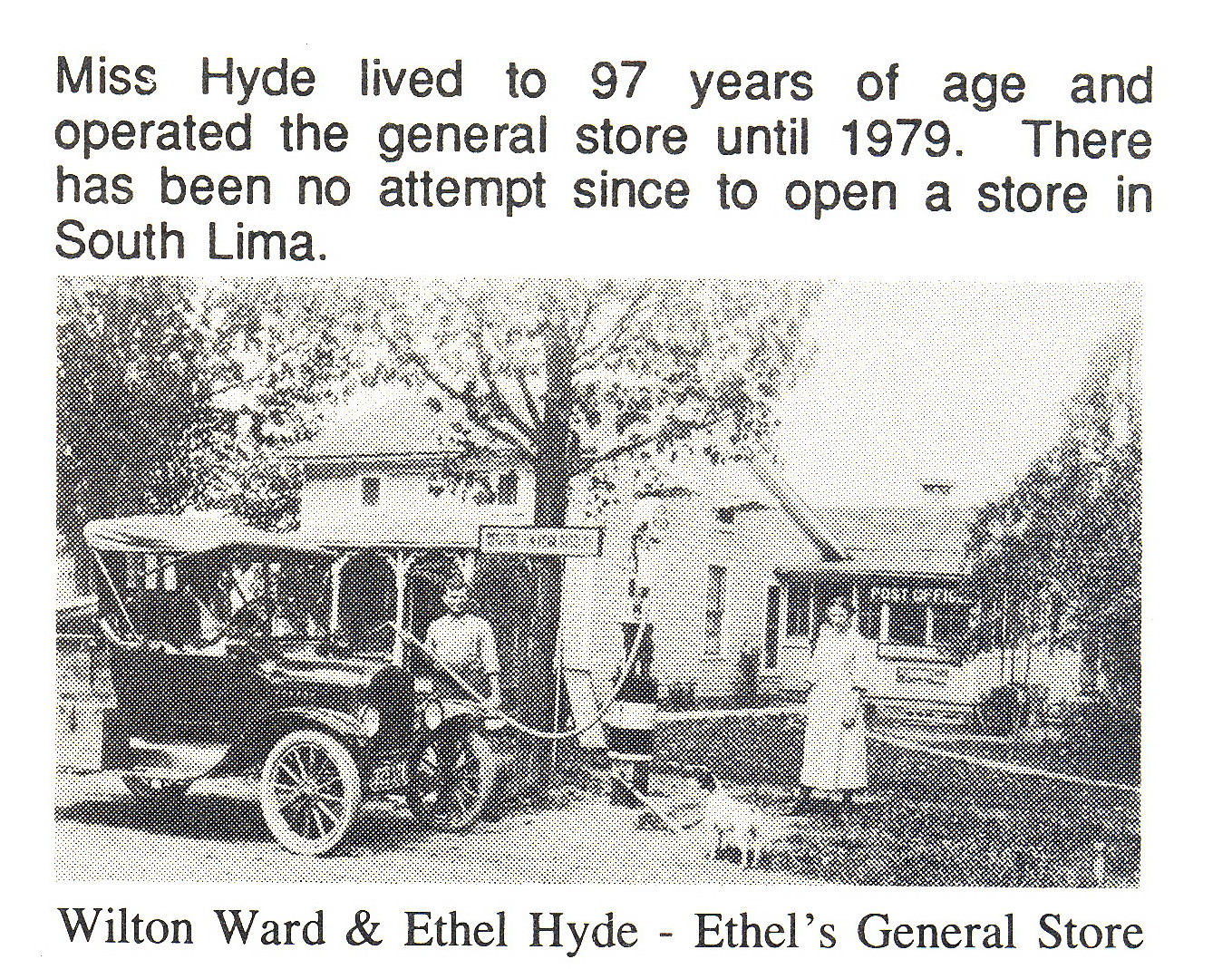The sepia-toned photograph, seemingly derived from a newspaper clipping, showcases a nostalgic scene from yesteryear. Central to the image is a quaint post office flanked by lush trees, emblematic of a simpler time. Parked in front of the building is a vintage car, hinting at the bygone era the picture captures. Positioned prominently are a well-dressed man and woman - Wilton Ward and Ethel Hyde - standing side by side, presumably engaged in conversation. The woman, Ethel Hyde, is noted for her remarkable longevity, having lived to the age of 97, and her steadfast dedication to running the general store until 1979. Since then, no effort has been made to reopen the store in South Lima. The bottom half of the photograph is textually adorned with the names "Wilton Ward and Ethel Hyde - Ethel's General Store," encapsulating the essence of the community landmark and its storied past. The photo serves as a poignant testament to the endurance and eventual cessation of small-town commerce.